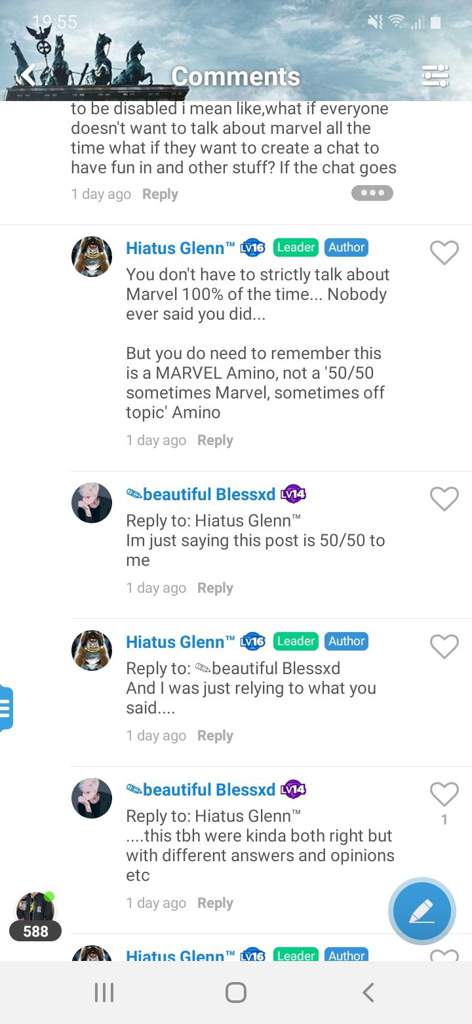A vibrant comment section unfolds on a website, evident from the dynamic exchange among users. At the top, a header showcases a picturesque blue sky dotted with a few clouds, beneath which majestically rise statues of gallant horses. The header is crowned with the title "Comments."

Below, the conversation ensues against a clean white background, with black text standing out clearly. Links within the text are highlighted in blue. Labels in green and blue designate "Leader" and "Author" roles, adding structure to the discussion. Each comment features a white heart with a gray outline on the right, providing a way for users to express their appreciation.

The visible discussion features a debate about the content focus of the community, marked by civil disagreements and clarifications. One user, possibly concerned about the community's flexibility, questions, "What if everyone doesn't want to talk about Marvel all the time? What if they want to create a chat to have fun in and other stuff?" Hiatus Glenn clarifies, insisting on the Marvel-centric nature of the space but allowing for occasional off-topic conversations.

Another user, BeautifulBlessed, shares their perspective that the focus feels split between Marvel and other topics. The dialogue continues, with Hiatus Glenn reiterating their point and BeautifulBlessed acknowledging the mix of opinions, saying, "we're kind of both right, but with different answers and opinions, etc." The conversation trails off with another reply from Hiatus Glenn, which is partially obscured at the bottom of the screen.